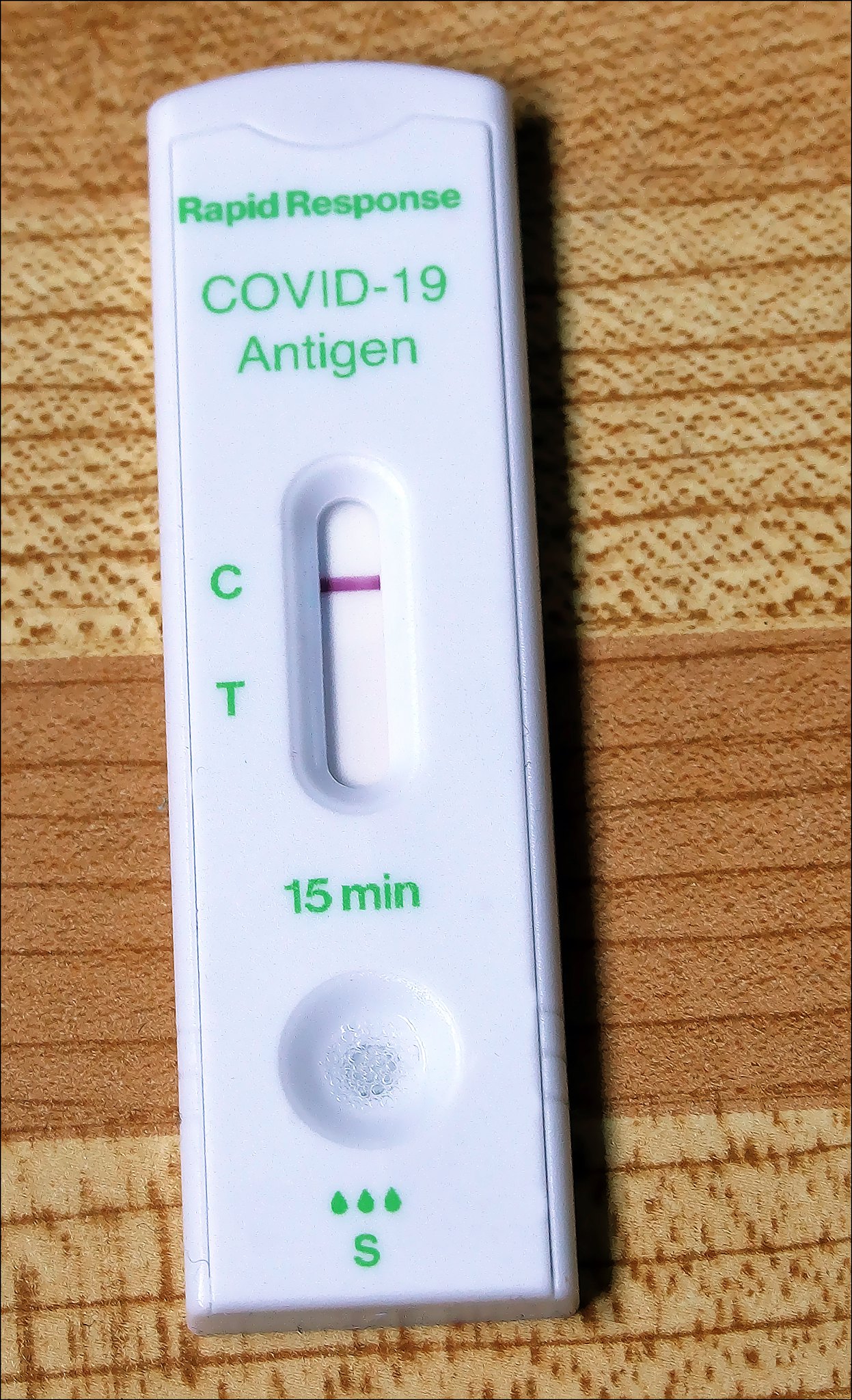The image displays a close-up of a COVID-19 rapid test kit placed on a textured, striped brown and golden surface. The test kit is white with text printed in green, which reads "Rapid Response, COVID-19 Antigen, 15 minutes." A long, oval opening is present at the top of the test kit, with a brown indicator bar visible within the opening. Beside the indicator bar, the letter "C" is marked in green. The textured surface beneath the test kit adds a distinct contrast, highlighting the importance and usability of the medical device for detecting the presence of COVID-19.